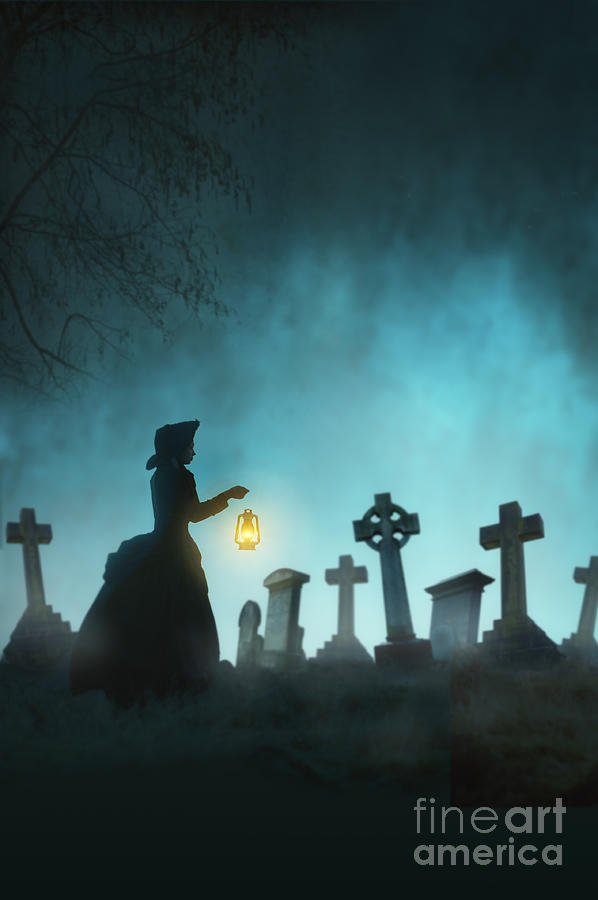This vertically aligned, computer-generated artwork depicts a haunting, late evening scene with a woman navigating a graveyard. The sky above transitions from a dark, almost black hue at the top to a charcoal gray, eventually blending into a blue tinged with clouds and smoke. On the left upper corner, a barren tree emerges, adding to the eerie atmosphere.

In the center stands the silhouette of a woman dressed in 19th-century attire, characterized by a bulky dress with a narrow waist and a bonnet on her head. She carries a lit, gold-glowing kerosene lantern in her right hand, which casts a subtle glow around her. She appears to be walking towards the right side of the image, through a cemetery filled with various grave markers. Among these, some are cross-shaped, while others are typical rectangular tombstones. One distinctive grave marker behind her sits atop a steeped podium with a cross at its peak.

A mist covers the ground, adding a spectral effect against the predominantly black earth. The lower right corner features the gray text "Fine Art America," indicating the artwork's origin.